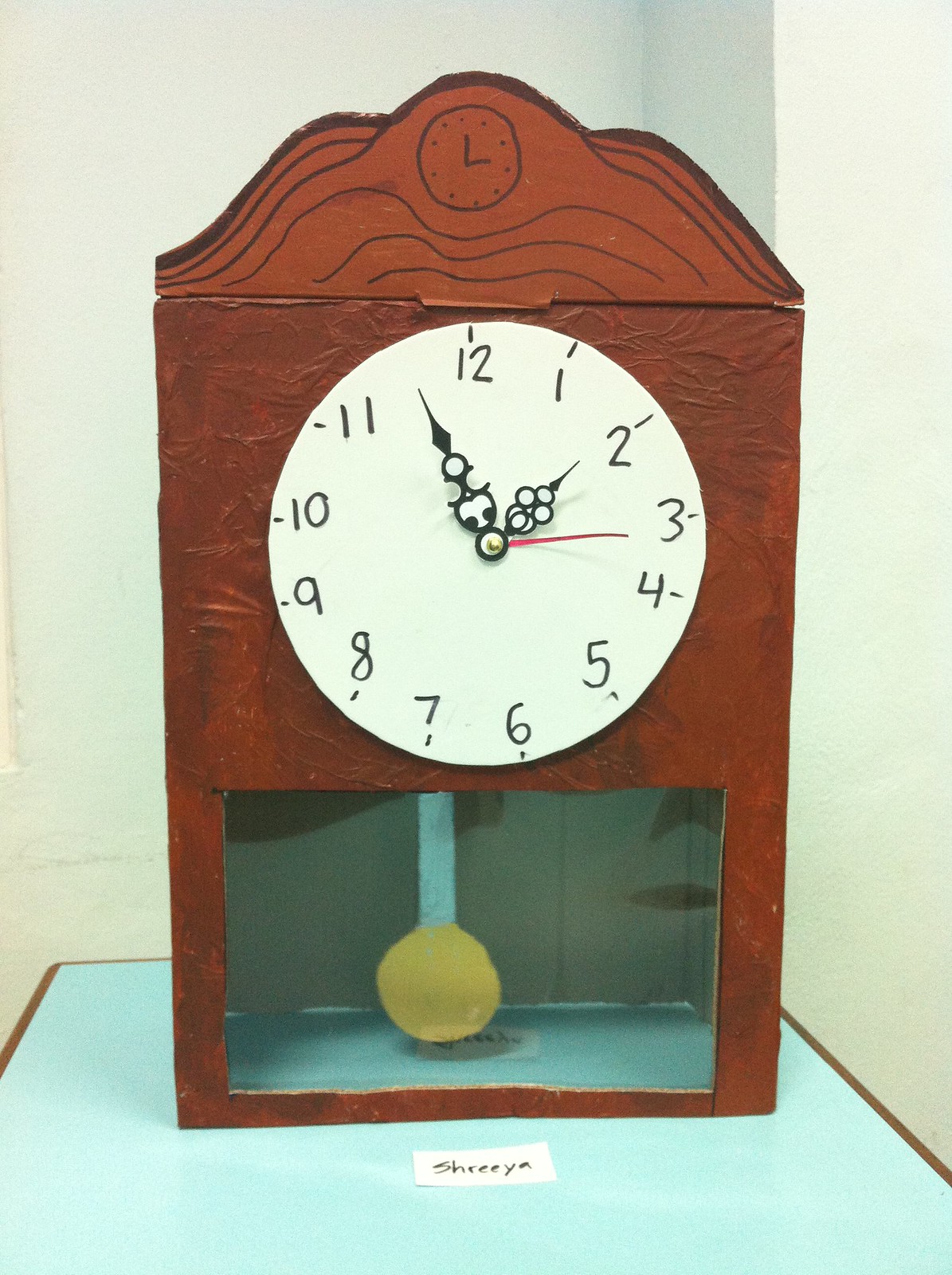This photograph captures a charming handmade cardboard clock, likely crafted by a child. The clock is placed against a white wall or corner, sitting on a light blue table with a subtle brown edging. A slip of white paper on the table bears the name "SHREEYA," indicating the creator.

The clock itself is constructed from cardboard and takes the shape of a vertical rectangle. The front appears to be painted, or perhaps a painted piece of paper has been adhered, as evidenced by some wrinkling which wouldn't typically occur with cardboard alone. A circular piece of poster board forms the clock's face. 

At the top of the face is the number 12, with the numbers 1 through 11 spaced around the clock face in an endearing, albeit imperfect, manner. Each number is accentuated with a small line, with no additional minute markers in between.

The clock features intricately made hands that resemble real clock hands: a large minute hand, a smaller hour hand, and a striking red second hand. The time displayed reads 1:53. Below the clock face, there is a horizontal rectangular cutout revealing a blue interior with a pendulum mechanism. The pendulum has a blue rod and a golden circular bob.

At the top of the clock, a decorative brown piece adds a whimsical touch with squiggly lines and another small clock drawn at the apex. This delightful creation showcases both creativity and skill, capturing the essence of a child's artistic endeavor.